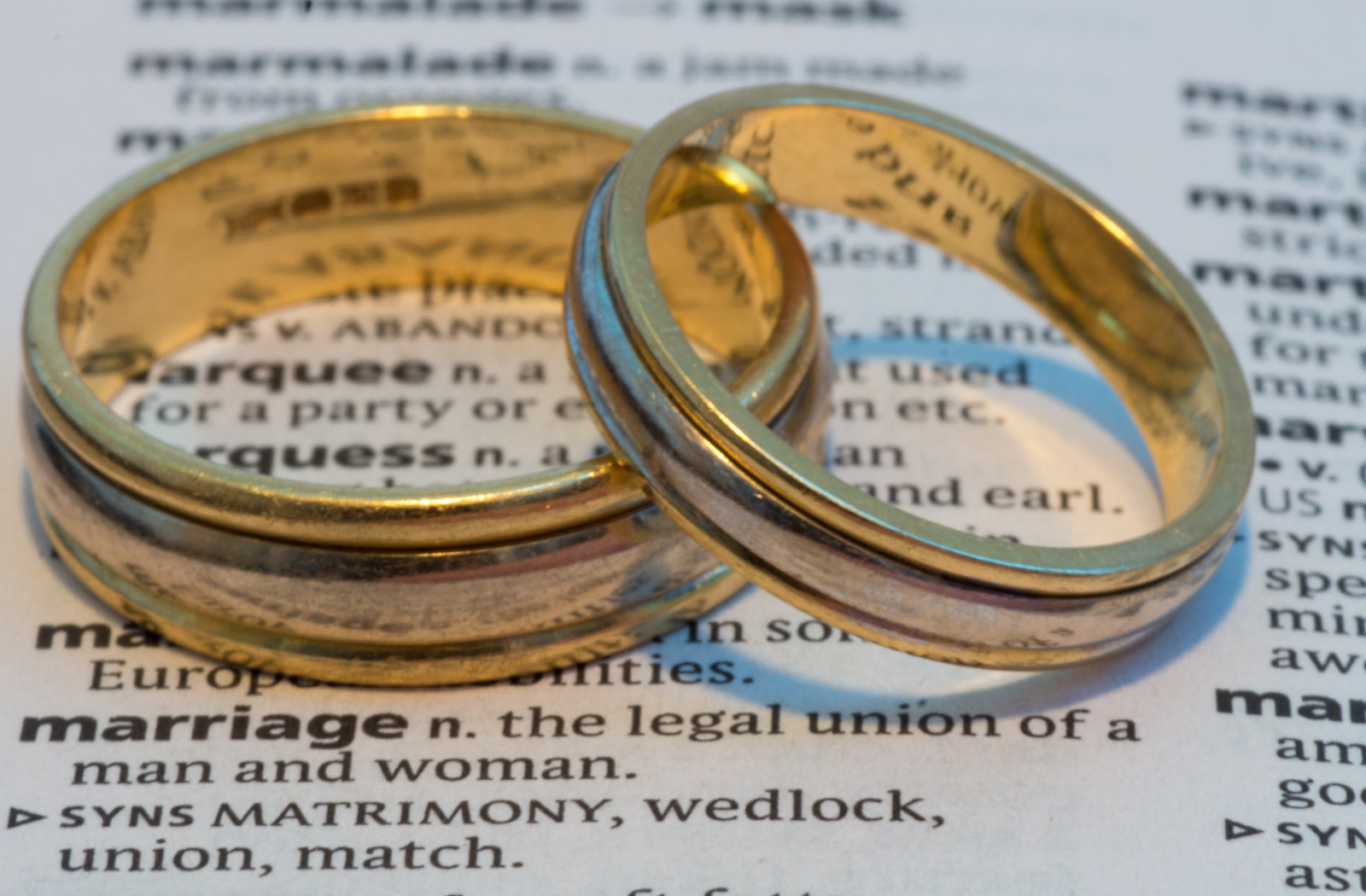This photograph showcases a pair of gold rings positioned together, suggesting they are part of a wedding set comprising a wedding ring and a wedding band. The wedding ring is notably thicker, while the wedding band is comparatively thin. Both rings feature intricate ridged designs. They are notably placed atop an open dictionary page, aligning them with a clear definition of the word "marriage" in black text, which states: "Marriage (noun): the legal union of a man and woman." The juxtaposition of the rings and the definition emphasizes the traditional symbolism and significance of marital commitment.